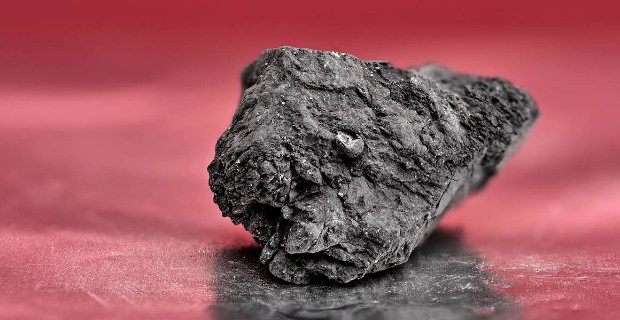The image is a close-up of a jagged, gray rock that resembles a piece of coal, with a dark, partially glossy surface. The rock is placed on a slightly reflective, rose-colored background that blurs towards the edges. The uneven surface of the rock shows varying thickness, thicker on the left and narrowing to a point on the right, featuring cracks and white, ashy mineral deposits. Shadows and reflections of the rock are visible on the rose surface, enhancing the contrast between the dark, charcoal-like rock and the red background. Some whitish-brown dust appears beneath the rock, possibly from the mineral deposits. This distinctive image is reminiscent of a lump of coal, similar to what might be shown to children during Christmas time for misbehaving.